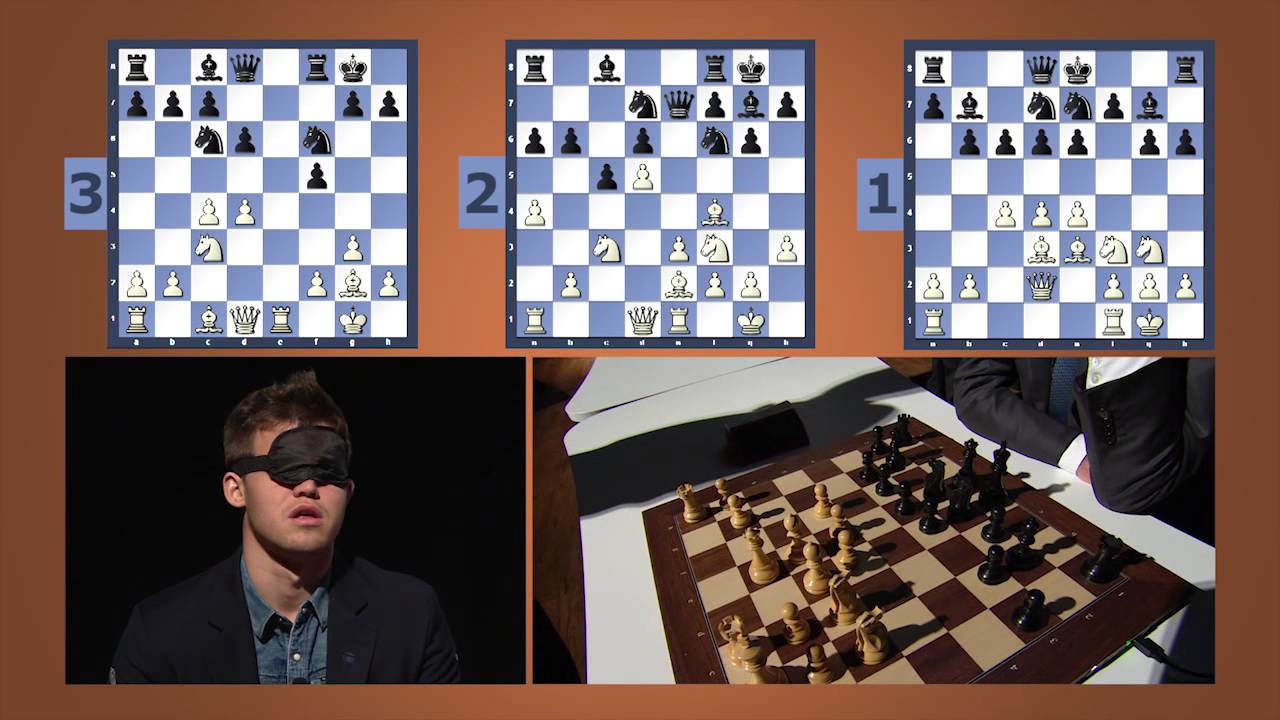The image depicts an intense chess scenario against a brown backdrop. At the top of the image, three electronic display screens show sequences of chess moves, labeled 3, 2, and 1 from left to right, each on a blue and white chessboard. The screens are bordered in dark blue, and the chess pieces on these boards are classic white and black. In the lower left corner, a young white man with short hair, dressed in a dark jacket over a blue jean shirt, is blindfolded as he participates in the game. He faces slightly to the right. On the bottom right, there's a traditional chessboard with brown and tan squares, placed on a white table, accompanied by a partially visible player. The board is set with standard white and black chess pieces, with white pieces on the left and black on the right, indicating an ongoing or about-to-start game. The scene captures the tension and complexity of a chess match, highlighting the variety of visual elements including color contrasts of black, white, beige, brown, blue-jean blue, and mahogany.